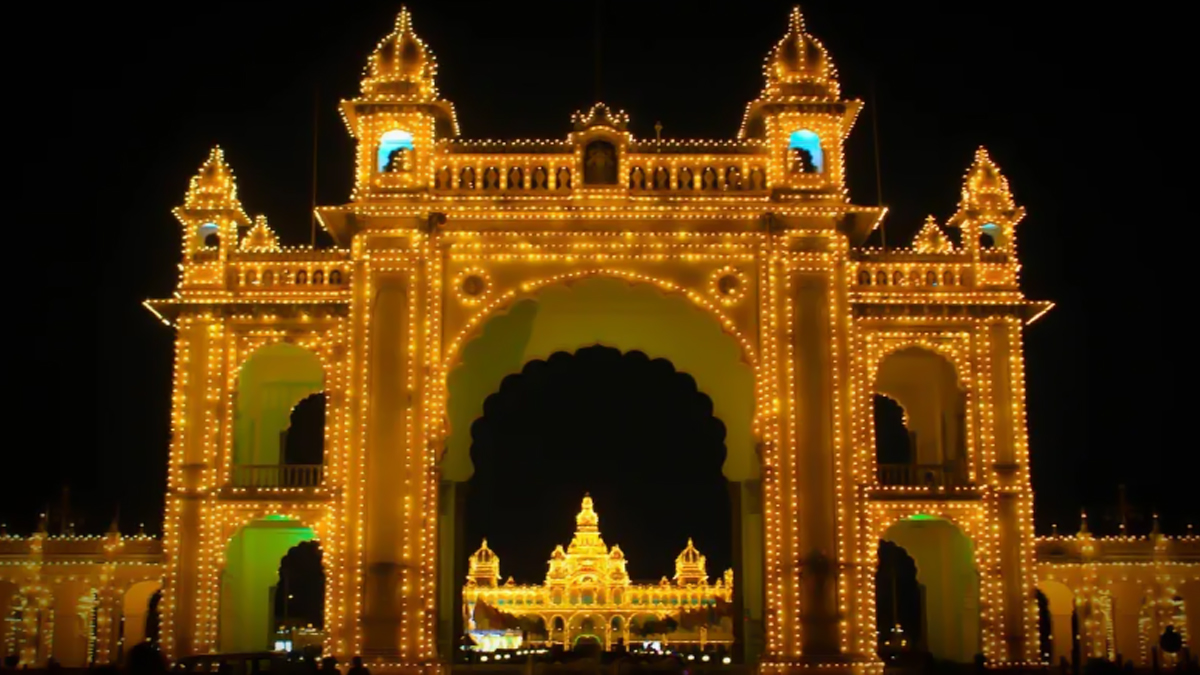This nighttime photograph showcases a majestic gateway leading to an illuminated palace, displaying a rich blend of Islamic architectural influences. The dark, starless sky serves as a dramatic backdrop to the scene. At the forefront, a grand archway bathed in gold and brown light forms the centerpiece, flanked by two-story rooms on each side, with tiny arches adorning a lower wall that stretches outwards. The gateway frames a pathway that leads to a distant palace, glowing in warm golden-yellow hues. The intricate structure is adorned with decorative spires, which are topped with twinkling blue and green lights, resembling fairy lights. The buildings' borders are meticulously outlined with bright yellow lights, enhancing the enchanting ambiance. The scene, devoid of any visible people, conveys a tranquil and captivating atmosphere, inviting viewers to marvel at the architectural beauty and its luxurious illumination.